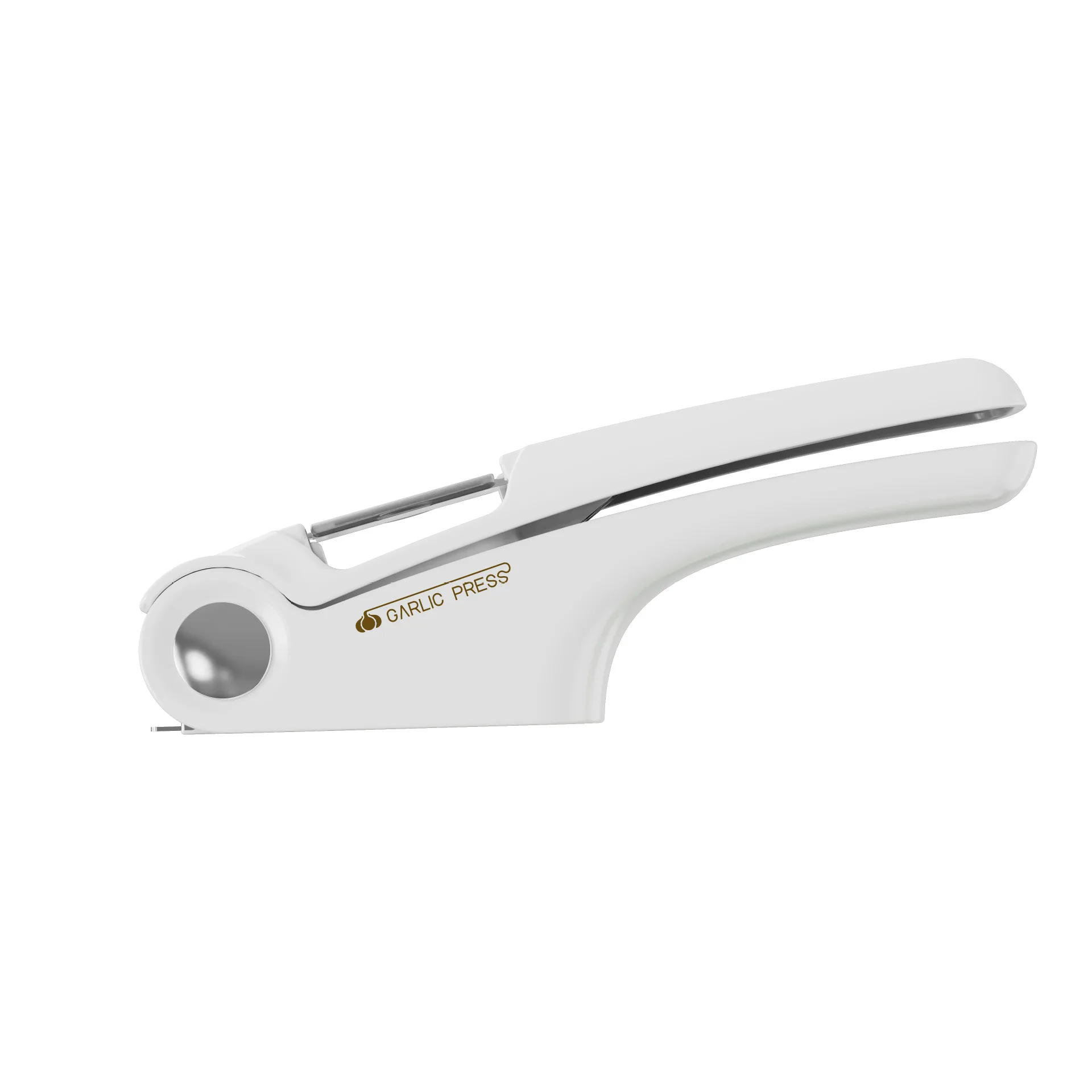This image features a white garlic press set against an entirely white background. The garlic press resembles a cross between a bird beak and a stapler, with two handles hinged together, allowing the top handle to lift and press down. There is a silver screw at the hinge, contributing to its functionality. The garlic press has a rectangular cutout that adds to its unique aesthetic. On the left side of the tool, printed in gold uppercase letters, it says "GARLIC PRESS," with a small illustration of a split garlic head above the text. The overall design is sleek and modern, giving it an unconventional appearance compared to traditional garlic presses.